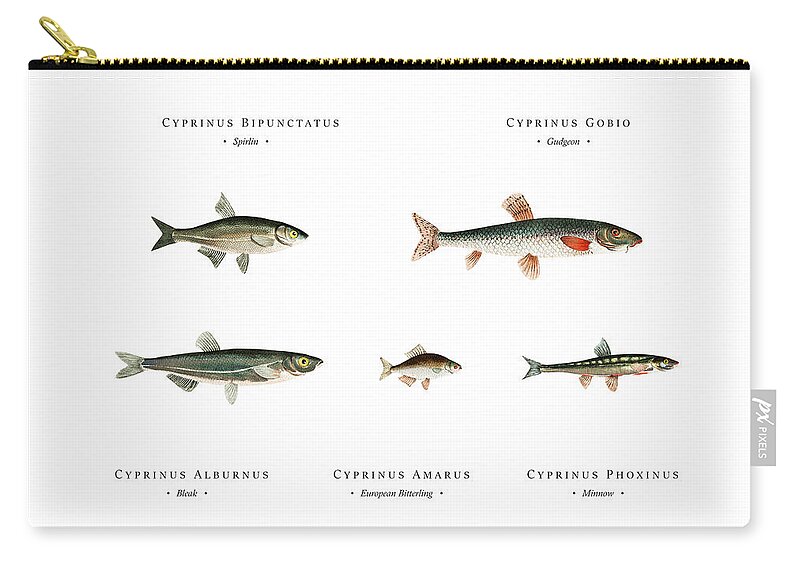This product image features a detailed view of a white zippered pouch, which could be used as a pencil case, makeup bag, or coin purse. The pouch is made of a rough-textured material and prominently displays a tag at the bottom right corner that reads "PX pixels." The zipper runs across the top of the pouch, featuring black fabric around it and a zipper pull that appears to be gold or brass colored. 

The design on the pouch showcases five painted illustrations of fish, each bearing scientific names: Cyprinus Bipunctatus, Cyprinus Gobio, Cyprinus Alburnus, Cyprinus Amarus, and Cyprinus Phoxinus. The fishes are of varying sizes, arranged with two on top and three below, and the names are written neatly beneath each illustration. The background color of both the pouch and the image itself is white, highlighting the detailed and realistic renderings of the fish.